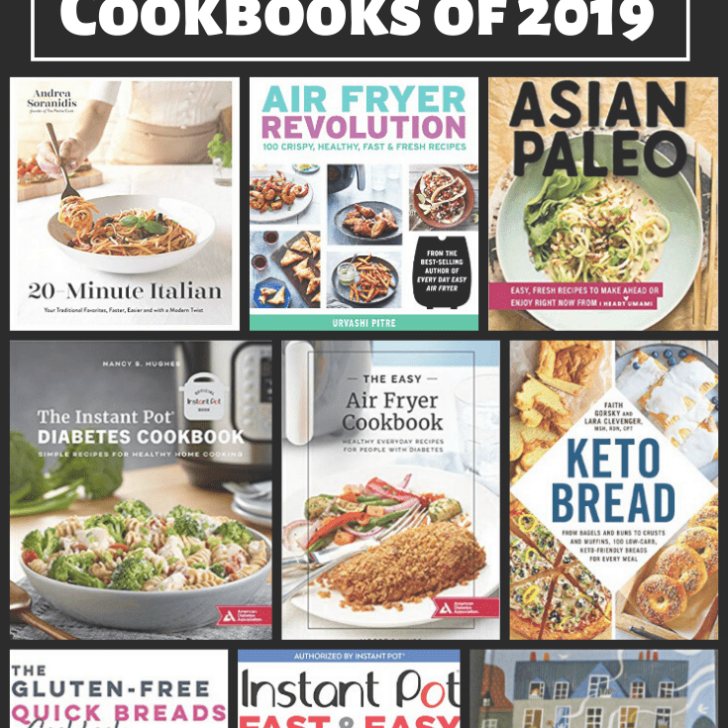This image is a cropped screenshot titled "Cookbooks of 2019," featuring nine thumbnails of cookbook covers. Arranged in three rows of three against a black background, the title at the top is partially cut off, making "Cookbooks of 2019" only partially readable within a white outline box. This appears to be a social media graphic, perhaps from Pinterest.

In the first row, the leftmost cookbook is titled "20-Minute Italian." Next to it, the middle thumbnail is "Air Fryer Revolution," and the rightmost cover is "Asian Paleo." 

The second row begins with "The Instant Pot Diabetes Cookbook" on the left, followed by "The Easy Air Fryer Cookbook" in the center, and "Keto Bread Cookbook" on the right.

In the third row, the top halves of the covers are visible, with the bottom halves cropped out. The leftmost thumbnail shows "The Gluten-Free Quick Breads," the middle cover reads "Instant Pot Fast and Easy," and the rightmost thumbnail is cut off, leaving only the top of a house visible without any readable text.